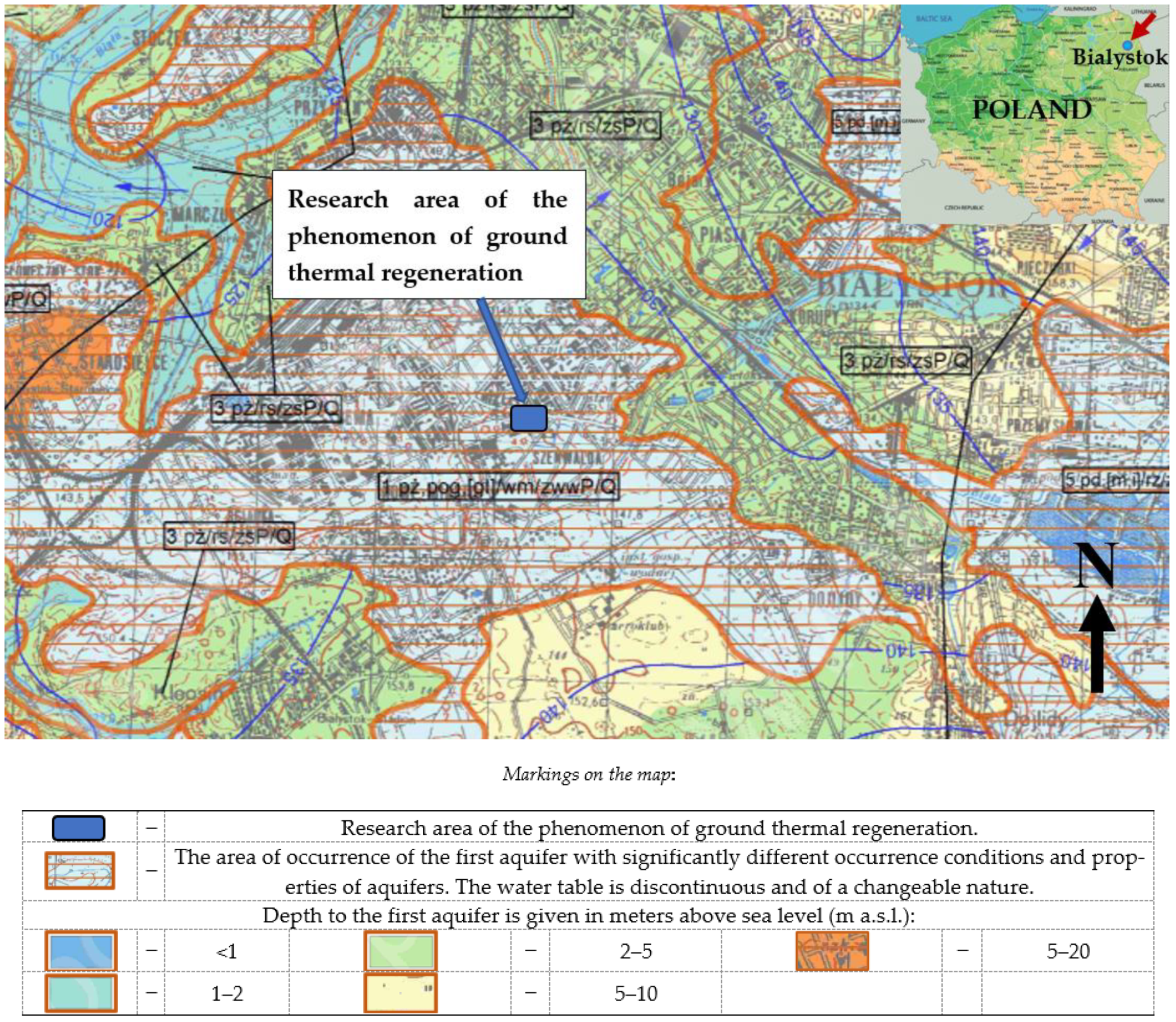This image is a detailed, colorful map of Poland, prominently featuring varied hues of green, yellow, orange, and blue. The top right corner confirms its focus on Poland, with specific mention of Bialystok highlighted by a blue circle and a red arrow. The map's central area contains a white box with the label "Research Area of the Phenomenon of Ground Thermal Regeneration," connected by a blue arrow to a blue box in the legend at the bottom. The legend clarifies this marking and others, noting the presence of areas with diverse aquifer conditions. The text in the white box elaborates that these areas reflect "the occurrence of the first aquifer with significantly different occurrence conditions and properties of aquifers," explaining that the water table is discontinuous and changeable. The legend also provides a color-coded guide to the depth of the first aquifer, given in meters above sea level (MASL), with different colors indicating specific depth ranges, such as less than 1, 1-2, 2-5, 5-10, and over 10 meters above sea level. Detailed sections labeled with numbers and letters, along with text that may either be in a different language or coded, enrich the map's scientific and geographic information.